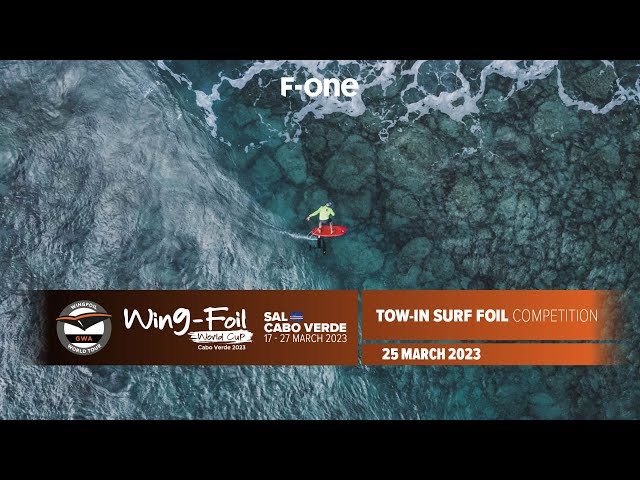The image portrays an aerial view of a vibrant body of water with various shades of teal, white, and black. At the center, a surfer maneuvers across the waves, amidst a setting dedicated to water sports competitions. Bold text spans the visual, announcing several events: the "Wing Foil World Cup Cabo Verde 2023" to the left and "Tow and Surf Foil Competition 25th of March 2023" on the right. Additional details specify "Sal Cabo Verde 17 to 27 March 2023" and the presence of the "GWA Wing Foil World Tour." At the top, "F1" is prominently displayed in white. The backdrop bursts with hues of blue, green, red, and orange, with water appearing almost liquid and dynamic, capturing the intense and colorful spirit of the competition.